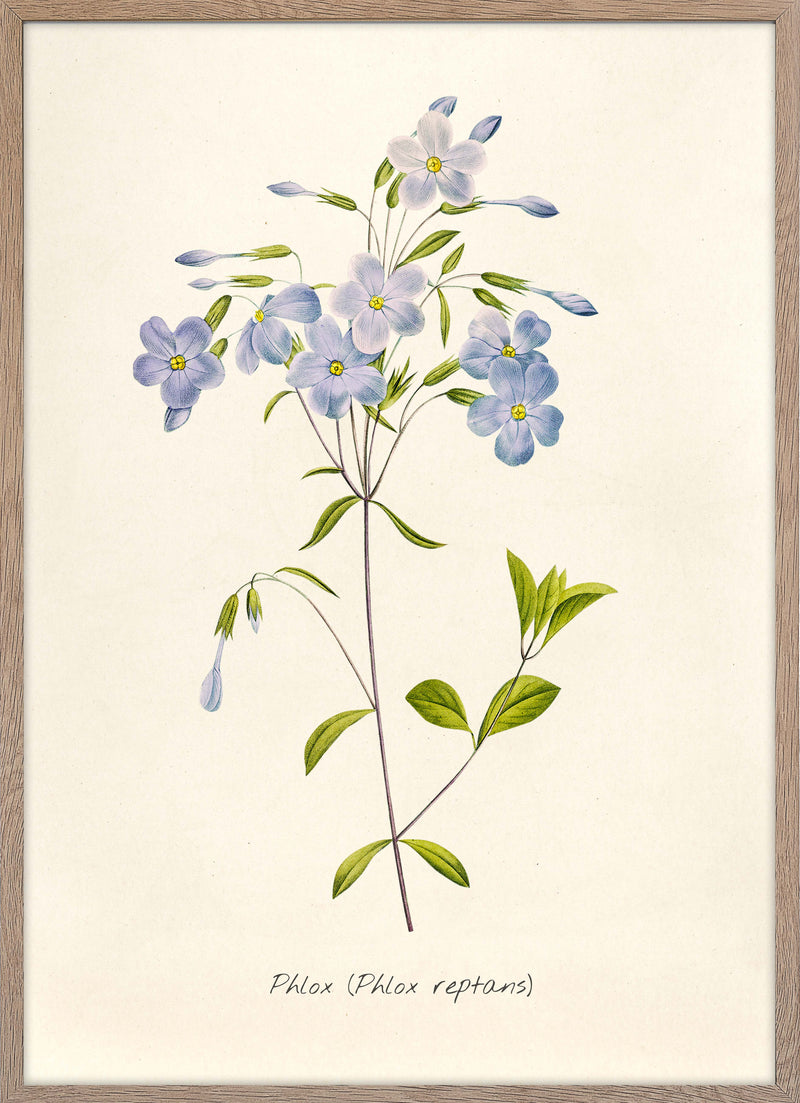This image showcases a delicate drawing encased in a light, thin frame. The artwork is rendered on an eggshell-colored paper or canvas, lending it a soft, vintage aesthetic. The focal point of the drawing is a cluster of bluish flowers, prominently positioned at the top. These blooms appear to sprout in abundance from the top of a slender, singular stem. A secondary, thinner branch emerges from the right side of the main stem, adding a subtle complexity to the composition. At the bottom of the image, the word "floats" is inscribed, possibly hinting at a title or theme for this ethereal depiction.